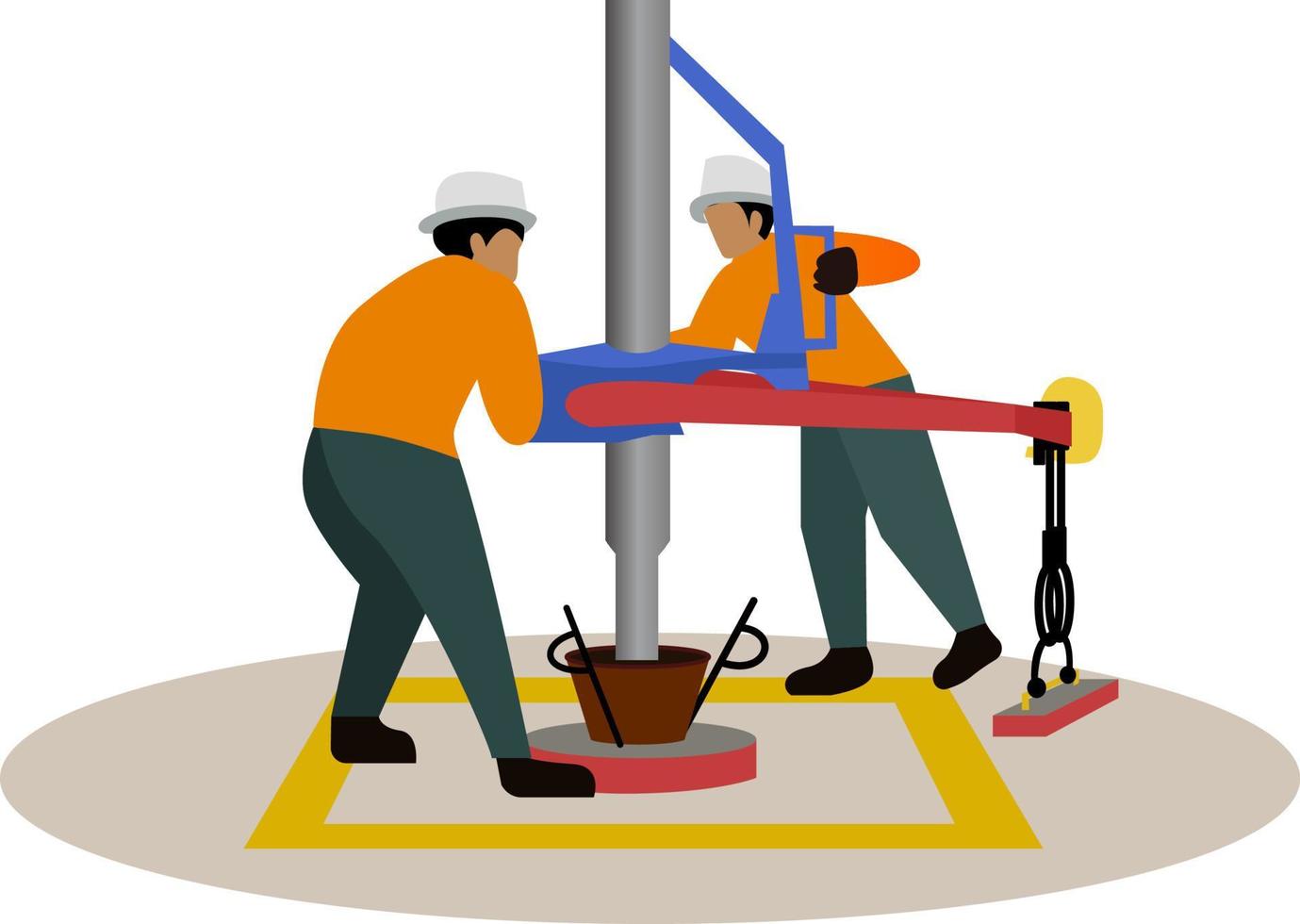This detailed illustration appears to be a computer-generated image or artwork depicting two construction or factory workers with tan skin and black hair, both wearing white hats and long-sleeve orange shirts. The workers are also donning gray pants and black shoes, along with black gloves. These figures, which lack facial features, are positioned around a vertical silver metal pole. One of them is grasping a blue handle, which is part of a large machinery apparatus that includes blue and pink components and is anchored by a red circle with a brown bucket at the base. The machinery also has an arm extending from it, featuring a plank attached to a rope. The workers are standing on a beige or white circular platform with an outlined yellow square, and the background includes black shapes and a brick at the bottom. The flat, felt-like design of the illustration suggests it may serve as artwork or a conceptual safety poster for factory operations.